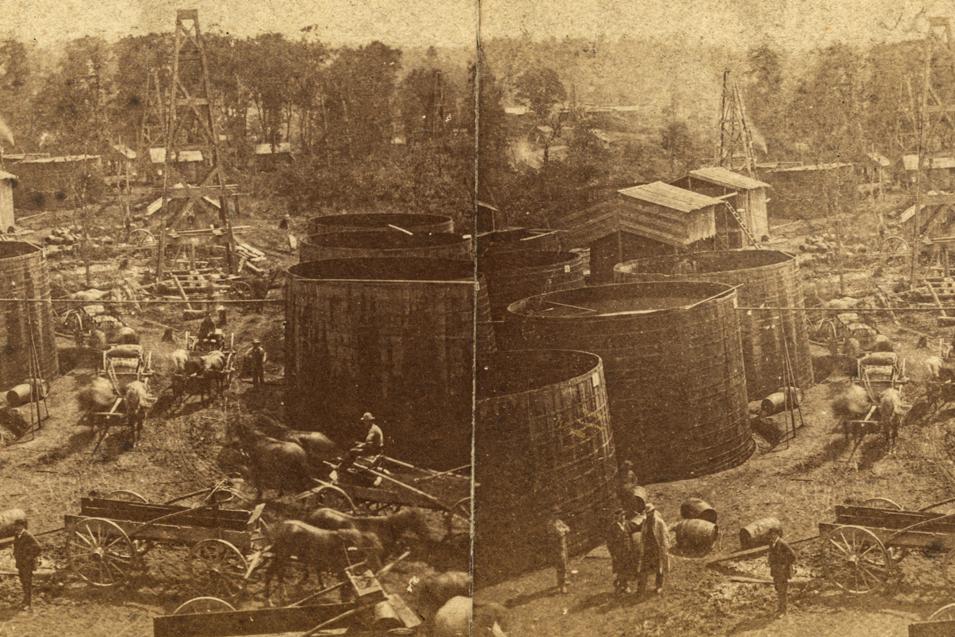This is a sepia-toned, black and white photograph, possibly resembling a vintage postcard, presented in two side-by-side images that capture different parts of the same scene. The setting is a bustling, old-time industrial area with a dirt road running through it. Wooden structures dominate the landscape, including large cylindrical vats bound with metal and several tall wooden oil derricks. The road is busy with numerous horse-drawn carriages, each with large wheels, transporting various goods. Scattered around are wooden barrels and other containers. The scene features men in old-fashioned attire, wearing long jackets and hats, indicative of the period. The background includes additional wooden buildings and a few standing trees. The overall quality of the image is low, with a distinctive yellow and black hue, enhancing its vintage feel.